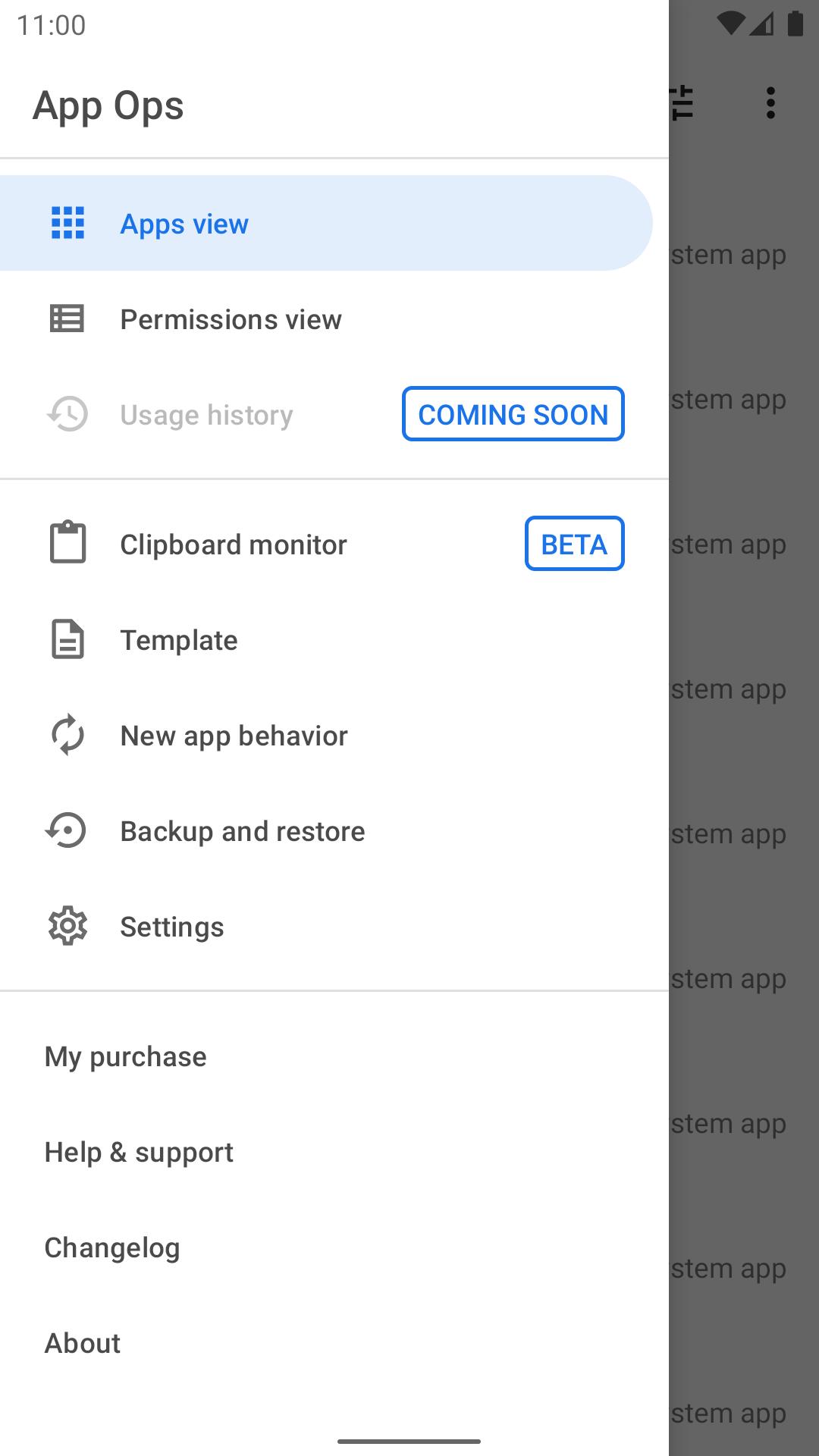This image displays a detailed screen from an application titled "App Ops." The display time in the top-left corner shows 11:00. The primary section features a list of categories with a white background and black text. The categories are arranged in the following order from top to bottom: 

1. "Apps View" (highlighted in blue)
2. "Permissions View"
3. "Usage History" (marked as coming soon)
4. "Clipboard Monitor"
5. "Template"
6. "Nice App Behavior"
7. "New App Behavior"
8. "Backup and Restore"
9. "Settings"
10. "My Purchase"
11. "Help and Support"
12. "Change Log"
13. "About" at the very bottom.

Adjacent to this list, on the right side of the screen, there's a holographic gray background running top to bottom, depicting a partial phone screen. The phone screen displays the text "S-T-E-M" and the word "App" repeated nine times. In the upper-right corner of the phone screen are several icons: a black cell phone signal, a Wi-Fi symbol, a connection icon, and a battery indicator.